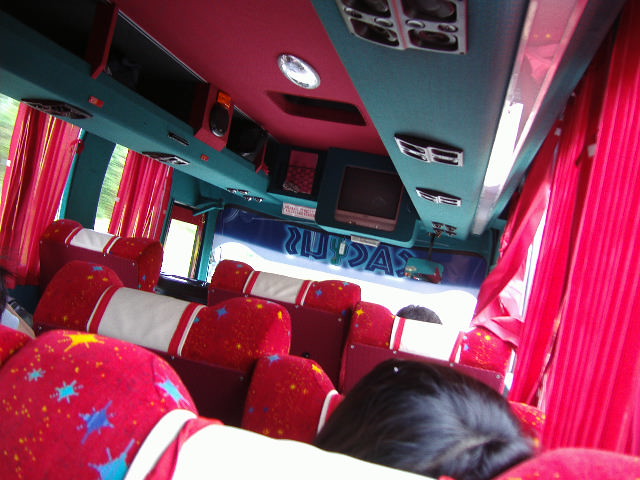The image captures the interior of a tour bus, taken from about three rows back, looking towards the front. The seats in the bus are a vibrant red, adorned with sparkly blue stars and numerous smaller golden specks. Each seat headrest is topped with a white cloth featuring red stripes. Bright pink curtains flank the windows, complementing the red seats and continuing the cohesive color scheme. The ceiling of the bus is red, while the upper section, which houses air conditioning vents and individual reading lights, is a teal blue. Two passengers are visible — one right in front with brown hair, and another farther up towards the front, also with brown hair. The sunlight streams through the front windshield, illuminating the interior. Partially visible near the front is some mirrored lettering, potentially on the bus's sunscreen, though it is difficult to decipher.